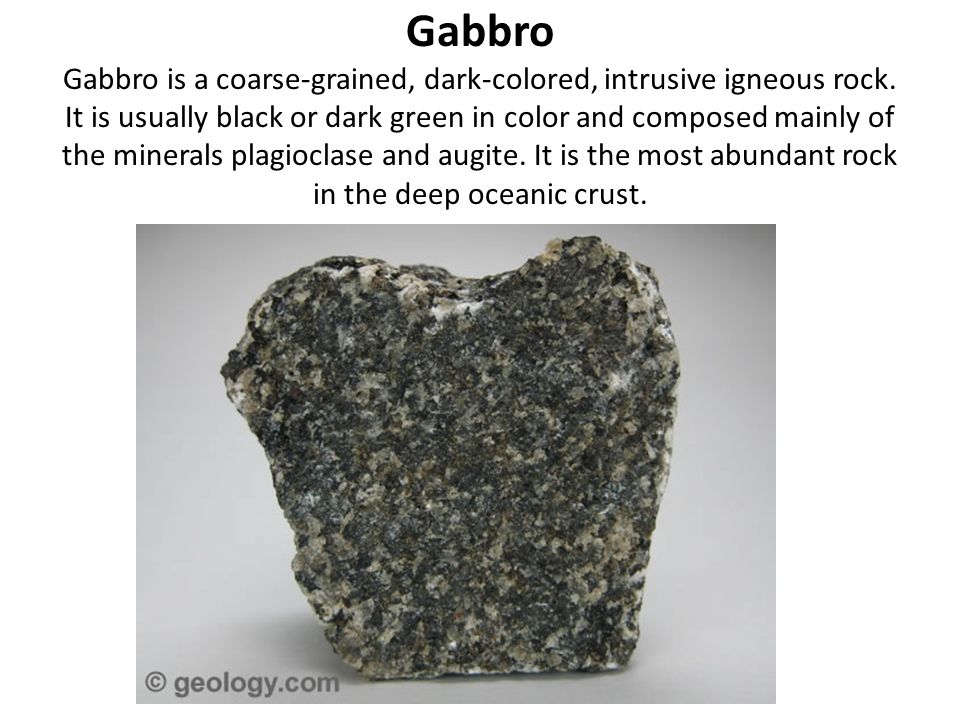The image displays a large rock specimen identified as Gabbro, a coarse-grained, dark-colored, intrusive igneous rock. The top of the image features text that reads "Gabbro," followed by a detailed description: "Gabbro is a coarse-grained, dark-colored, intrusive igneous rock. It is usually black or dark green in color and composed mainly of the minerals Plagioclase and Augite. It is the most abundant rock in the deep oceanic crust." The Gabbro sample shown is mostly black and gray, with speckles of white or beige, and has an almost square shape. The background of the image is gray, with no additional objects present. The bottom left corner notes the source of the image, geology.com.